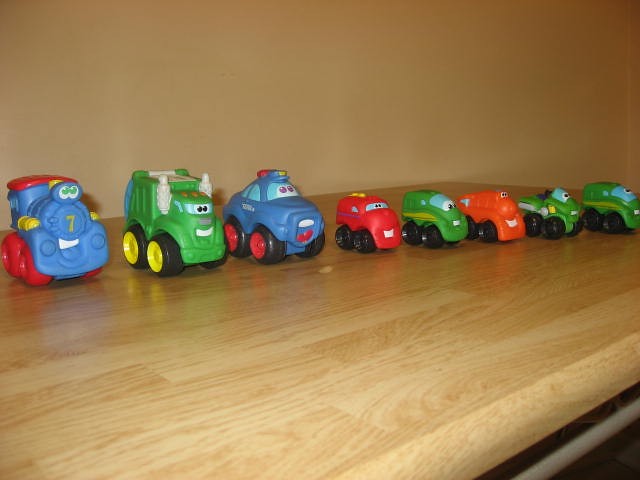This image shows a collection of eight toy vehicles meticulously arranged on a shiny, light-colored wooden shelf against a beige tan wall. The toys are positioned from left to right in decreasing size. The first vehicle is a blue train bearing the number one, characterized by its toy design and friendly appearance. Next is a green truck with smiling features, black wheels, yellow rims, and wing-like protrusions on either side. The third vehicle is a blue police car with distinct red rims, a playful red tongue, white teeth, and a light bar on its roof. Following that is a red car adorned with two small yellow buttons on top. Subsequently, a green car with yellow side stripes appears, followed by a smiling orange-red car displaying white teeth. Near the end of the line is a unique green toy resembling a motorcycle. Finally, the sequence concludes with a green and yellow van. Each vehicle is equipped with cheerful eyes and a grille-like mouth, adding to their whimsical charm.